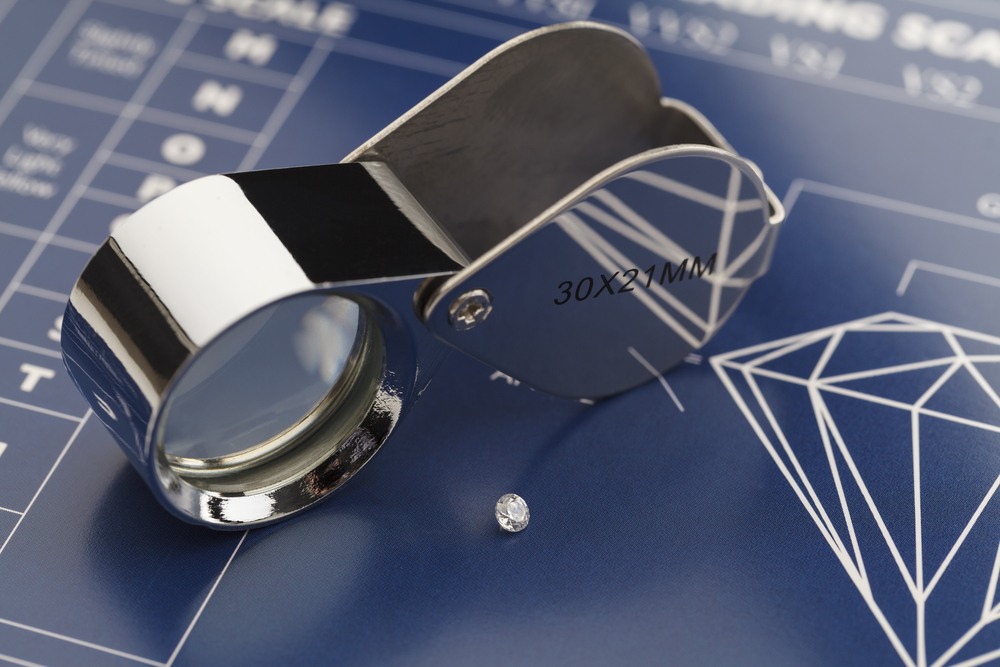This close-up photograph features a jeweler's loupe and a small diamond positioned on a dark blue background with a grid pattern and various white markings reminiscent of a blueprint, including a white line drawing of a diamond in the bottom left corner. The jeweler's loupe, which is teardrop-shaped and made of reflective silver, possesses a circular magnifying lens that can swing outwards from its housing via a small screw hinge located at the corner. The magnification strength, "30x21mm," is inscribed in black on the loupe. The small, circular faceted diamond beside the loupe is crystal clear and shiny, further enhanced by the contrasting dark blue surface adorned with what appears to be a scale or measurement guides. The background also contains alphanumeric codes in grids, possibly representing different grades or sizes used in the evaluation of diamonds.